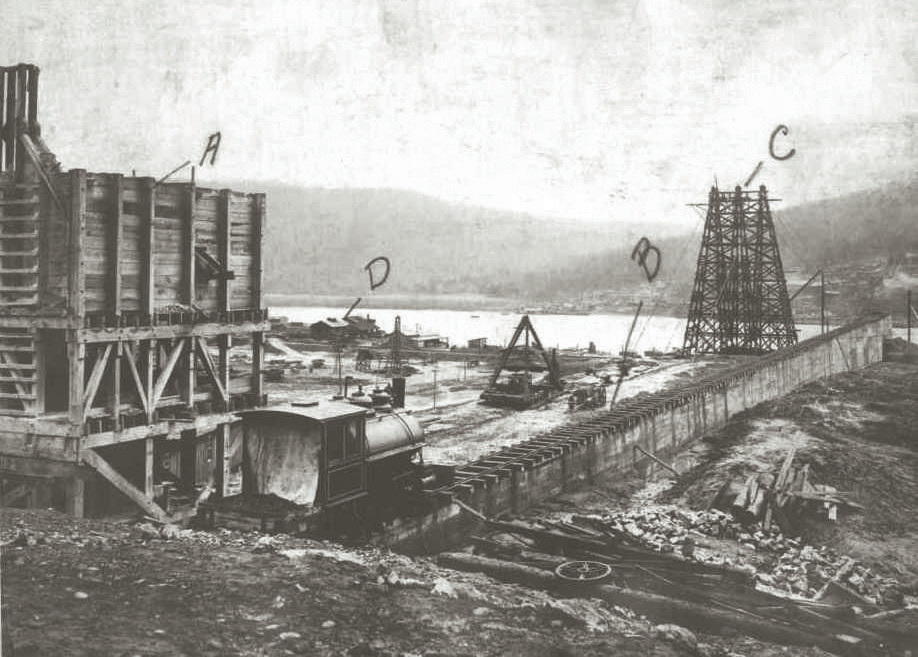This grainy black-and-white vintage photo captures a bustling construction site, likely from the early 20th century. The focal point is a multi-story wooden structure on the left, labeled "A" with a line pointing to it. Below it is a vintage train car, marked with the letter "D," situated on train tracks extending towards various distant buildings, suggesting this area might be under further construction. To the right, letter "B" points downward to more train tracks, indicating this could be related to the transportation system, possibly for a grain elevator or a dry dock. The right side of the image, marked with "C," highlights steel trellis-like structures that appear to be power lines or scaffolding, aimed towards the water in the background. Additionally, piles of rocks and other construction materials suggest ongoing heavy work. The distant hilly landscape and body of water could imply the potential construction of a dry dock or even a bridge. Pen markings on the image provide clues to the various points of interest, enhancing the historical and procedural context of this construction site.